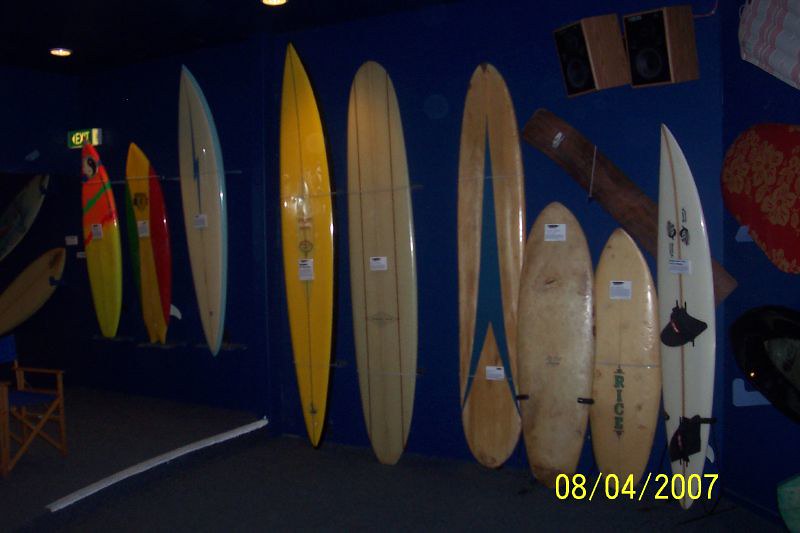This is a detailed color photograph capturing a collection of surfboards propped against a dark blue wall. The surfboards are arranged vertically as if standing. Starting from the left, there is an orange surfboard, followed by a green and yellow one, then a yellow surfboard with colors reminiscent of a banana split, a green, yellow, and red surfboard, a white surfboard adorned with a blue electric bolt, a beige surfboard, and a brown wooden surfboard featuring a blue chevron in its center. Additionally, there are two brown boogie boards and a white surfboard or paddleboard. The room is dimly lit, visible only by two ceiling lights and a faintly lit green exit sign in the distant corner, indicating it says "Exit" in white lettering. At the bottom right of the photograph, the date is stamped in yellow, reading 08-04-2007. No people are present in this image, which highlights the vibrant and varied surfboards against the contrasting dark blue background.